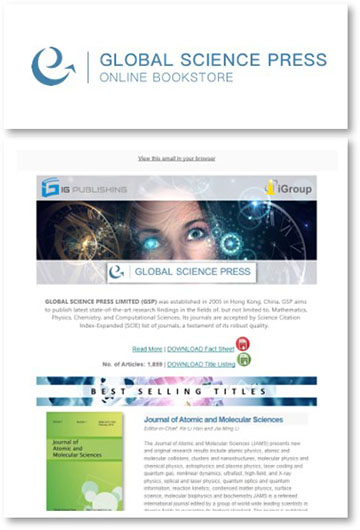The image depicts an article featured on a white background. The top section is enclosed in a slightly bordered white box, distinct from the lower portion. In the upper left corner of this box, there's a blue logo resembling a stylized letter "E" that tapers to a point, with the text "Global Science Press Online Bookstore" written below it.

Central to the image is a striking picture of a woman with one vivid blue eye, surrounded by bright blue circular patterns and elements resembling a clock face in the background. Below the image, the following text is displayed prominently: "IG Publishing, iGroup, Global Science Press, Global Science Press Limited (GSP) was established in 2001 in Hong Kong, China." Further down, options such as "Read more," "Download fact sheet," and "Download the listing" are presented, along with the metadata noting "Number of articles: 1,899."

Towards the bottom, the article references the "Journal of Atomic Molecule and Molecular Science" as one of the best-selling titles, accompanied by an image of a green book located to the left.